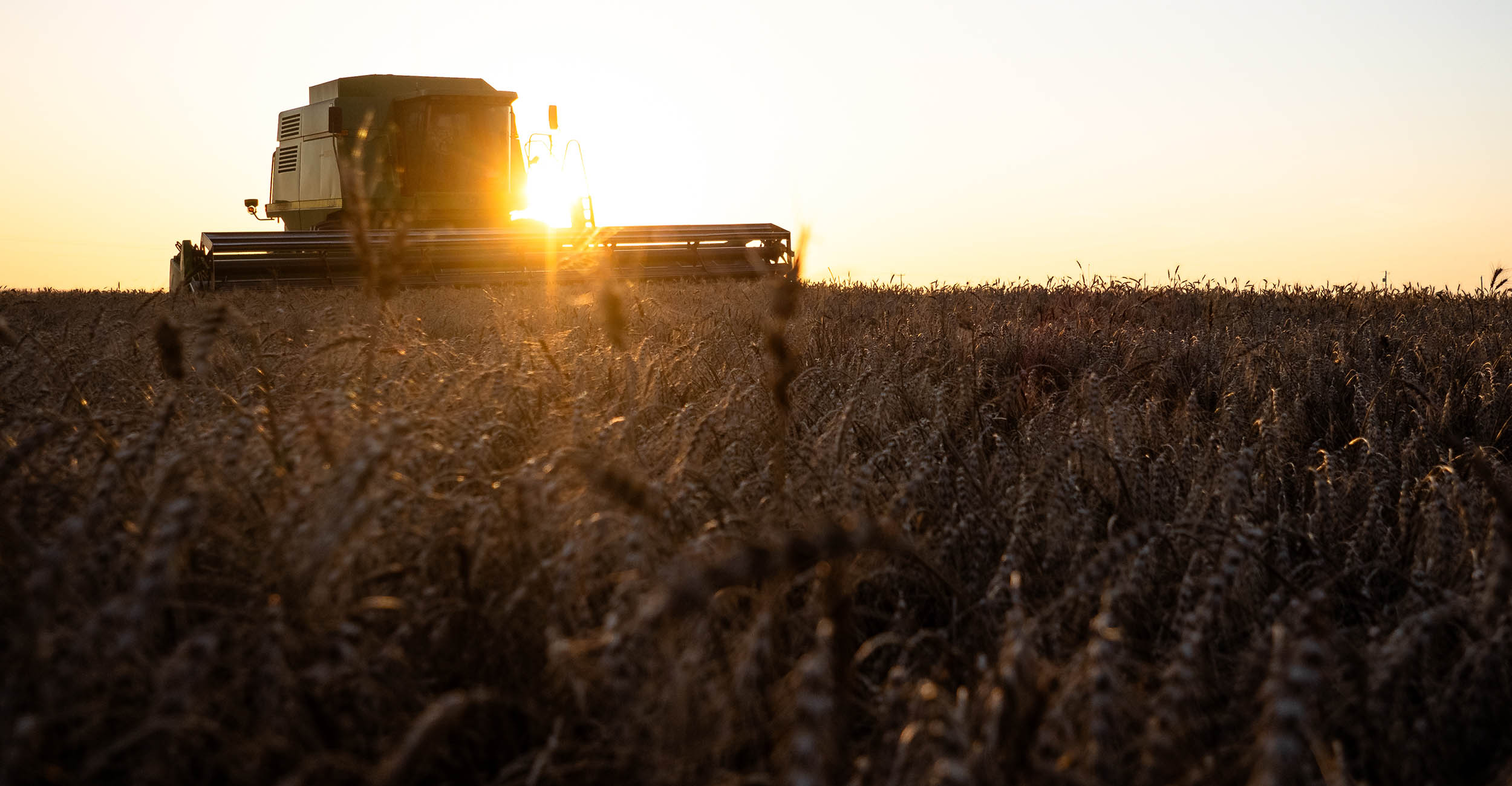The photograph showcases a vast wheat field bathed in the golden hues of sunrise or sunset. Dominating the left side of the image is a substantial piece of farm equipment, presumably a tractor fitted with a wide, boxy attachment designed for collecting or processing the wheat. The machinery, likely a wheat thresher, stands silhouetted against a clear sky with no visible clouds. Fields of wheat stretch across the image, from an enlarged, somewhat blurry foreground to more defined regions in the distance. The vibrant colors of the scene encompass shades of brown, yellow, gold, white, and black, encapsulating the essence of a peaceful, industrious farm atmosphere. The sun peeks just to the right of the machinery, casting a serene and almost painterly light over the whole scene, suggesting the quiet moments of dawn or dusk.